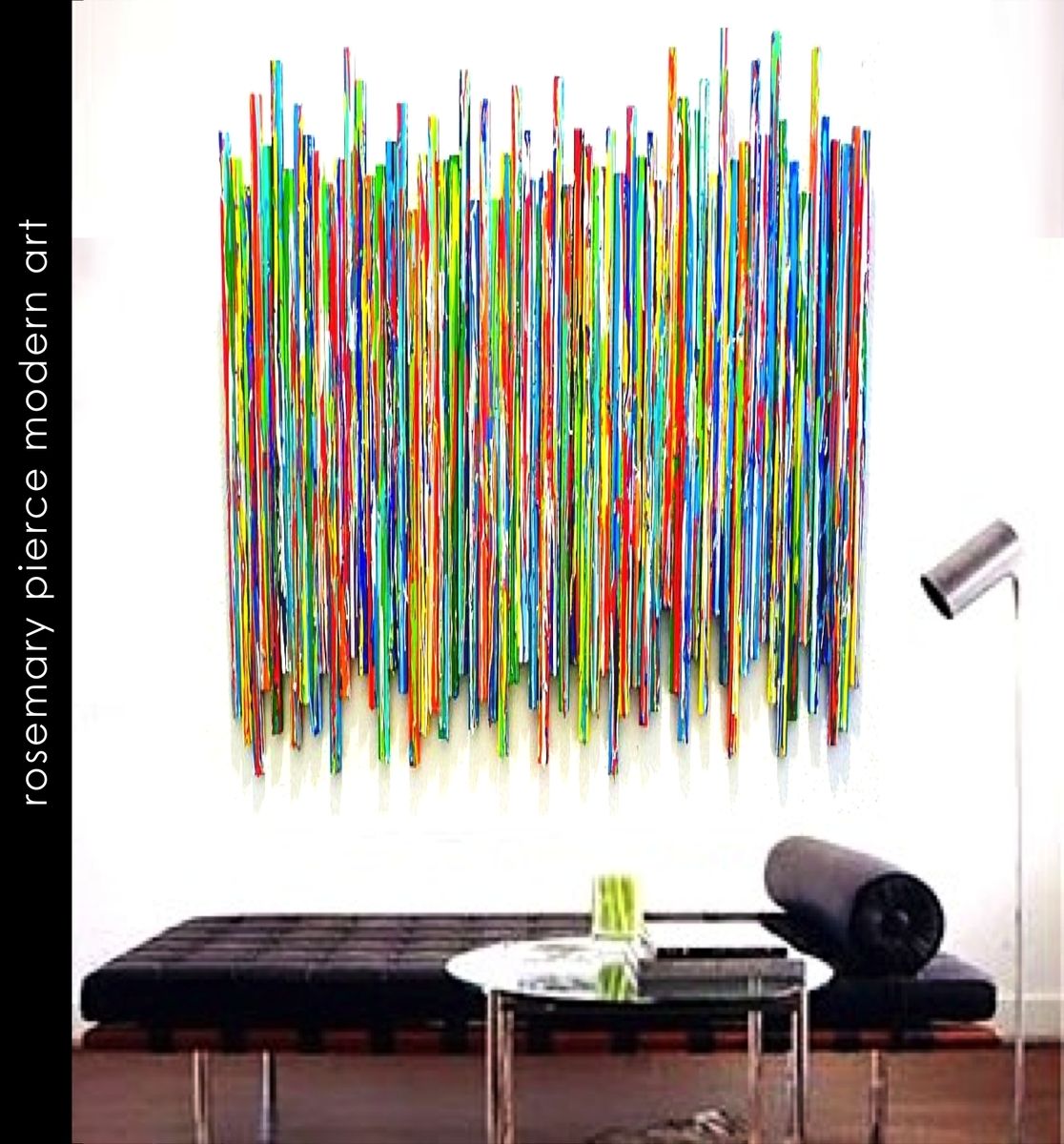The artwork displayed is a vibrant, multicolored installation mounted on a pristine white wall. The piece consists of numerous vertical lines, each of varying lengths, arranged closely together, creating an effect reminiscent of a condensed sound wave chart or a cluster of colorful popsicles. The palette spans the entire rainbow, with hues of greens, blues, reds, yellows, and oranges, forming a dynamic and engaging visual. Below this captivating artwork is a modern black leather bench, featuring sleek gold or rose gold legs. 

In front of the bench sits a glass-topped table, supported by legs that match the artwork's vibrant colors. On the table rest two coffee table books and another intriguing green object, adding to the setting's eclectic charm. To the right of the scene, a silver light fixture directs its glow downward, illuminating the area. On the left side, a black strip running down the wall bears the inscription "Rosemary Pierce Modern Art" in sleek white font, standing out against the dark background. 

The scene is anchored by a warm wood floor, adding a touch of natural elegance to the contemporary space.